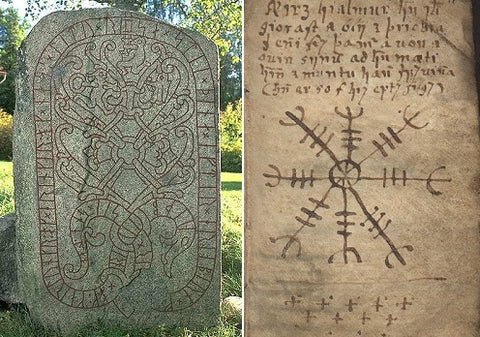The image is composed of two side-by-side photographs. The left photograph features a stone tablet positioned in a grassy, outdoor setting with rocks, trees, and a blue sky in the background. Engraved on the tablet is a line-drawing of a snake, starting from the bottom and spiraling around the stone, enclosing various runes spaced along its body. Additionally, the snake's tail loops around its head at the bottom, and inside the snake's coil, there appears to be an intricate design, possibly depicting figures or creatures, although the details are difficult to discern. The right photograph displays a piece of fabric or parchment covered in text written in a script that resembles Cyrillic or Mediterranean languages. In the center of this text is a circular symbol with eight radiating lines, each line adorned with three marks and ending in a moon-like curve with three prongs. Below this symbol are rows of small plus signs, with one row containing five plus signs and another containing four.